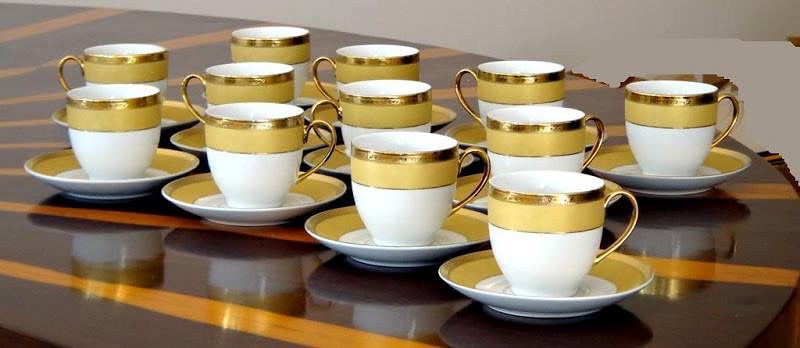In the photograph, a dozen teacups with their matching saucers are meticulously arranged on a round wooden table adorned with a glass protector. The table is crafted from dark brown wood and features an intricate starburst pattern, with orangish-yellow rays emanating from its center, enhancing its elegant design. Each vintage-style teacup stands out with a shiny gold gilt band encircling the rim, followed by a tan band midway down, and a white bottom. The handles of the teacups are also accentuated with gold gilt, providing a touch of opulence. The saucers mirror this pattern, featuring a gold gilt band on the edge, a tan band following it, and a white center, creating a cohesive and refined tea set display.